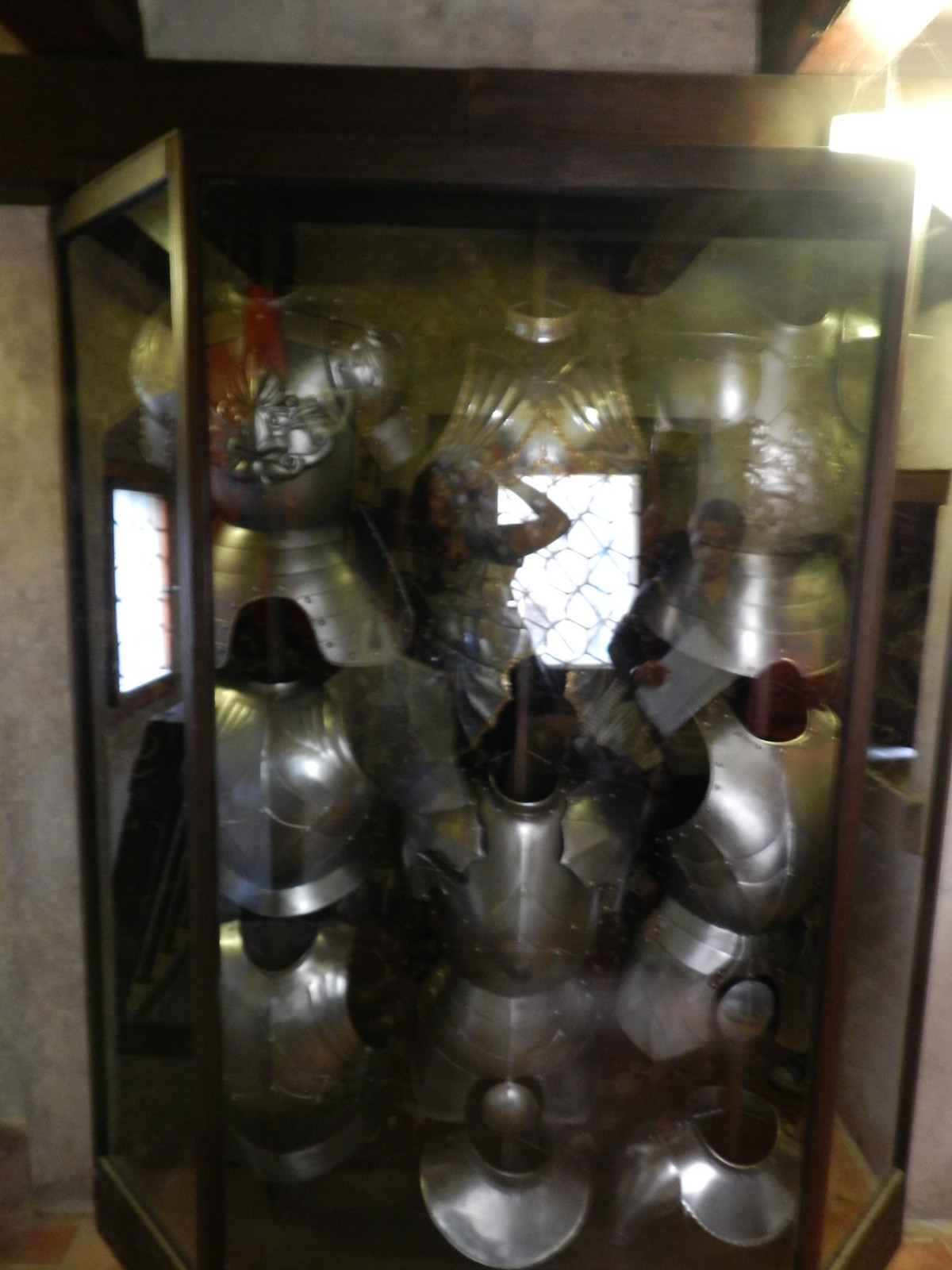The photograph showcases a large hexagonal glass display case, possibly situated in a museum, against a stone wall. The display case, framed in dark brown, almost chocolate-colored wood beams, houses nine pieces of gleaming, silver armor arranged in three rows of three. The armor pieces primarily consist of breastplates covering the chest and torso, along with waist armor that extends over the hips. No helmets or leg armor are visible. Reflections in the glass reveal the faint image of the photographer wearing a white shirt, with their arm centered in the frame as they hold up a phone or camera to capture the image. Additionally, the reflections display windows and a door, adding depth to the setting. The top of the case is framed by a white section or wall.